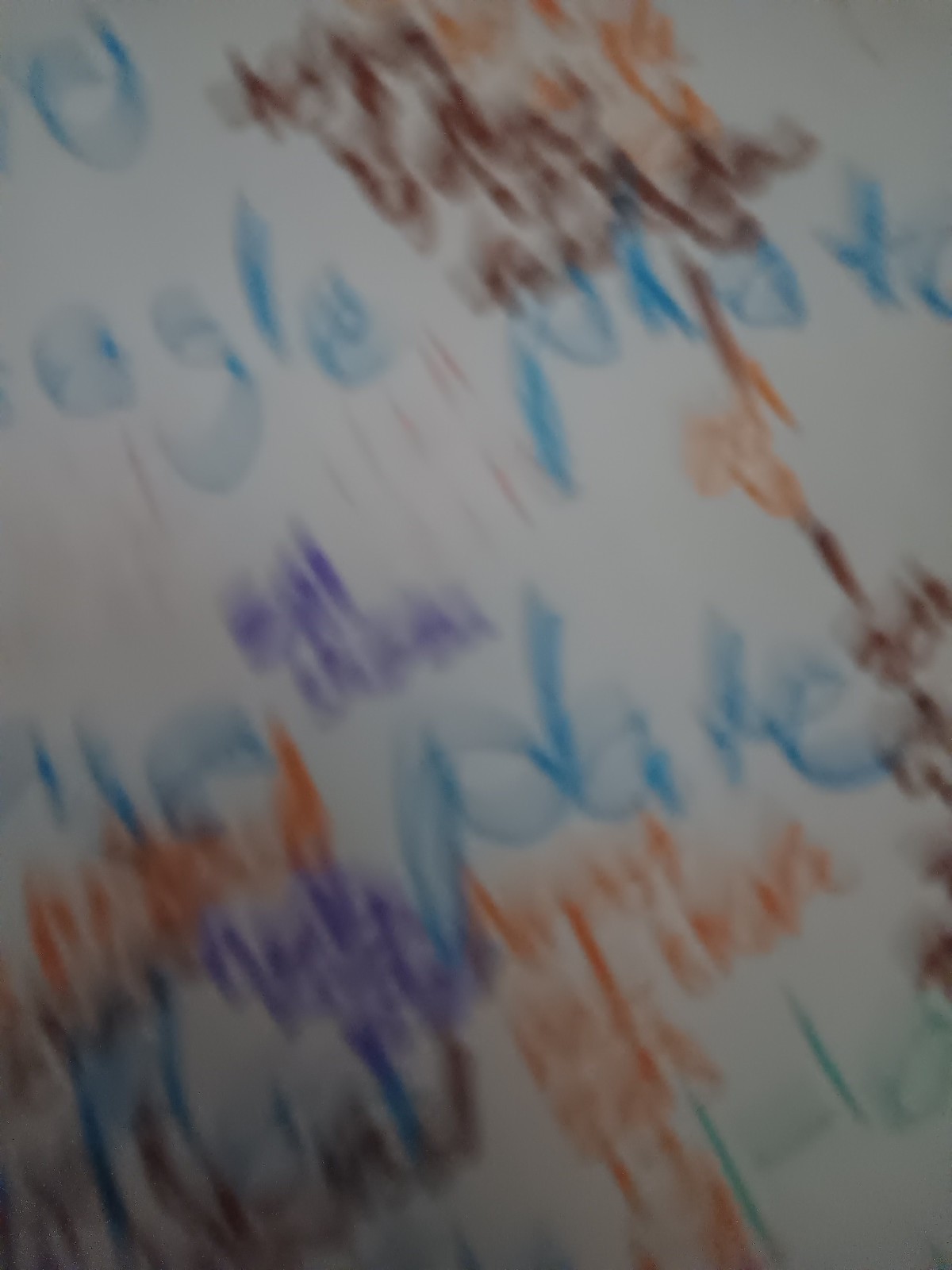A close-up color photograph captures a page filled with an array of handwritten words in various ink colors, including blue, purple, orange, green, and brown. The image is notably blurry, making the specific words difficult to decipher, though "plate" in blue ink is discernible in the center. The text seems to be segregated into clusters based on color, with brown and orange words grouped at the top, and a mix of purple, blue, and orange towards the bottom left corner. The overall effect is such that it's ambiguous whether the overlapping of words is due to the blurring of the image or if the words are actually written on top of each other. The arrangement of these colorful words hints at the possibility that a larger, coherent pattern or picture might emerge if the image was viewed from a distance.